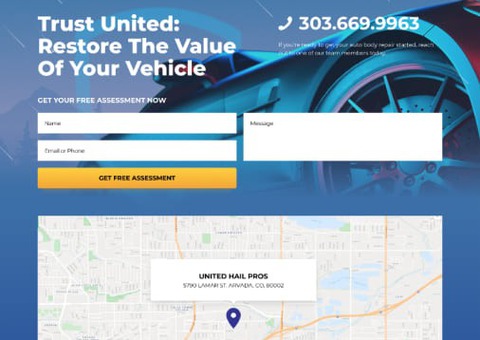The website for Trust United features a prominent header with the bold white text "Restore the Value of Your Vehicle" positioned in the upper left corner. On the right side, beginning near the center, there is a phone number displayed alongside a phone icon for easy contact. Beneath the main slogan, a smaller text reads "Get Your Free Assessment Now," suggesting immediate action. Below this, you can see a blurred long rectangular input box, likely intended for the user to enter their name. Another long rectangular input box follows but its contents are indistinguishable.

On the right, there's a larger box, roughly the size of both input boxes on the left combined, which likely contains a field labeled "Message." This section is intended for users to fill in their inquiry or details about their vehicle. The background image showcases a partial view of a car, notably the right tire and some of the side, which subtly fades into a blue tone. 

Towards the bottom of the page, a map highlights the location of United Hail Pros, with the text presented in black and accompanied by a location icon, providing a clear visual cue for the business's geographical area.